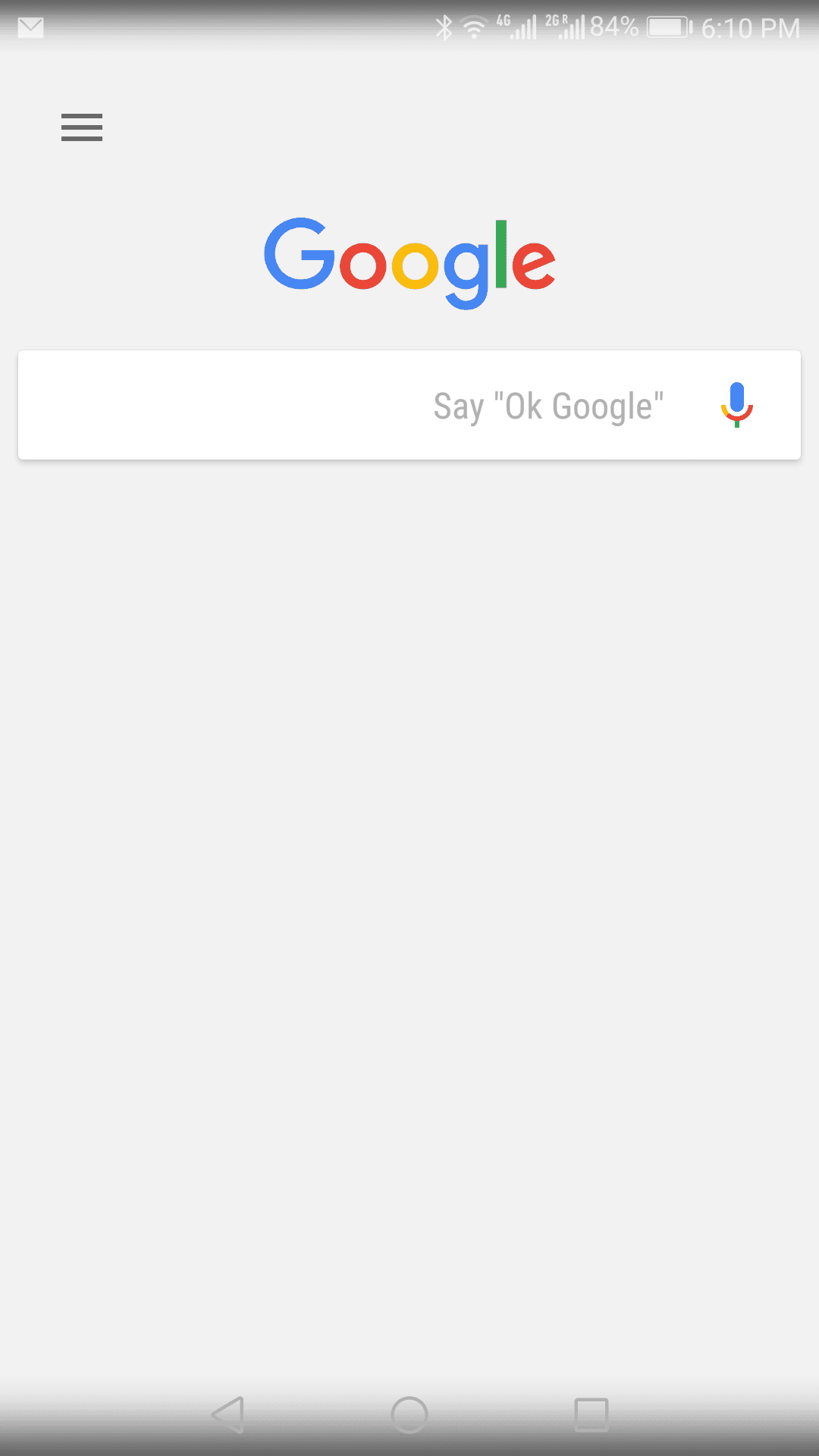This image is a simple screen capture from an iPhone displaying a Google search page within an app. At the top, the standard iPhone status bar is visible, showing the time as 6:10 PM, along with icons for battery life, signal strength, and upload/download activity.

Below the status bar is the familiar Google logo, which stands out with its multicolored letters: a blue 'G', a red 'o', a yellow 'o', a blue lowercase 'g', a green 'l', and a red 'e'. Beneath the logo, the search bar is prominently displayed, featuring the text "say (Ok Google)" in parentheses, and a microphone icon to the right—indicating that the voice search feature is active.

At the very bottom of the screen, there's a navigation bar with three standard symbols: a left-pointing arrow for 'Back', a circle for 'Home', and a square for 'App Switcher'. The background of the screen is primarily gray, giving a clean and uncluttered appearance, with no additional text or images visible. This setup suggests that the user has activated Google’s voice search feature and is ready to provide a voice command.

Overall, the image captures the essentials of the Google search interface on an iPhone, marked by its minimalistic design and functional layout.